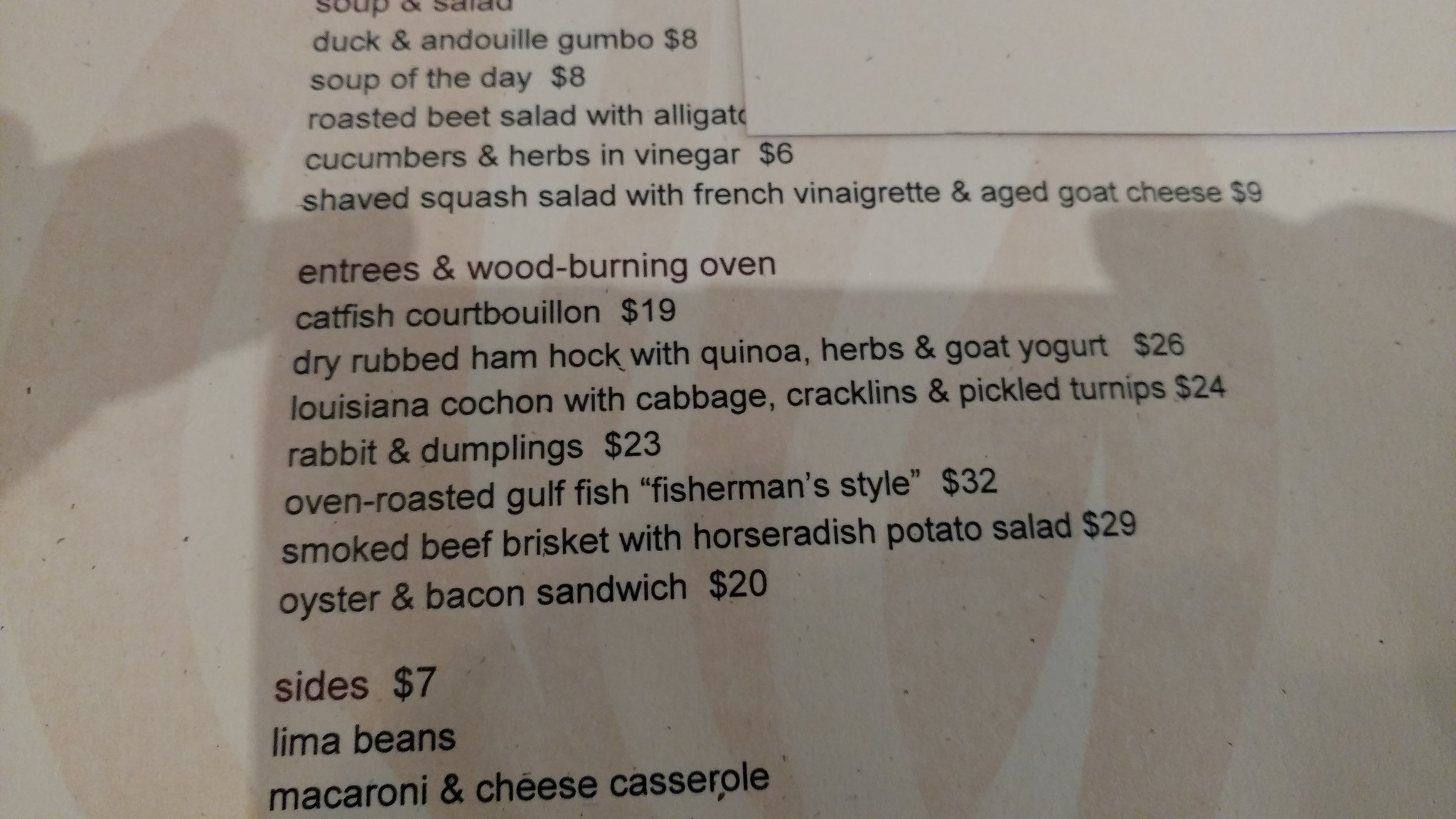A detailed image caption:

"A close-up shot of a portion of a white menu filled with various food items and their corresponding prices. The shadow of an off-camera person's hand is clearly visible on the menu. Listed among the appetizers are duck and gumbo for $8, soup of the day for $8, and cucumbers with herbs and vinegar for $6. Detailed entrees from a wood-burning oven feature prominently, such as dry-rubbed ham hock with quinoa, herbs, and goat yogurt for $26, Louisiana croissant with cabbage, cracklings, and pickled turnips for $27, and fisherman's-style oven-roasted Gulf fish for $32. Towards the bottom are sides priced at $7, including lima beans and macaroni and cheese casserole, with presumably more options below the visible portion. The top right part of the image is obscured by the edge of a white, rectangular card resting on the menu."